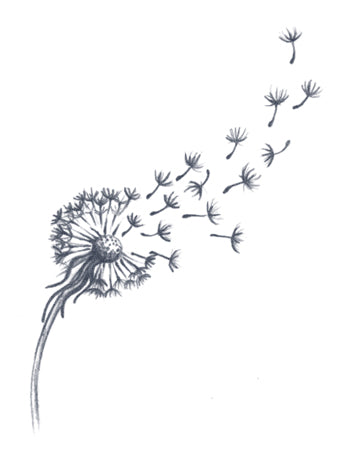This black and white sketch beautifully captures the delicate nature of a dandelion in transition. Starting from the bottom left, the stem emerges with a gradient from white at the base to a darker gray as it reaches the center of the flower. The flower's center, resembling a bulb, is detailed with black spots and fine hairs swirling downward. From this point, the image shows a dramatic scene where the feathery seeds, known as achenes, lift off and drift into the air. Approximately a third of these seeds are depicted mid-flight, with a trail starting from the cluster near the center and gradually thinning out as they ascend toward the top right corner. Some seeds remain attached, displaying the moment just before they too will be carried away by the wind. The sketch vividly showcases this ethereal process, emphasizing the flow of seeds that seem to dance upward, guided by an unseen breeze.